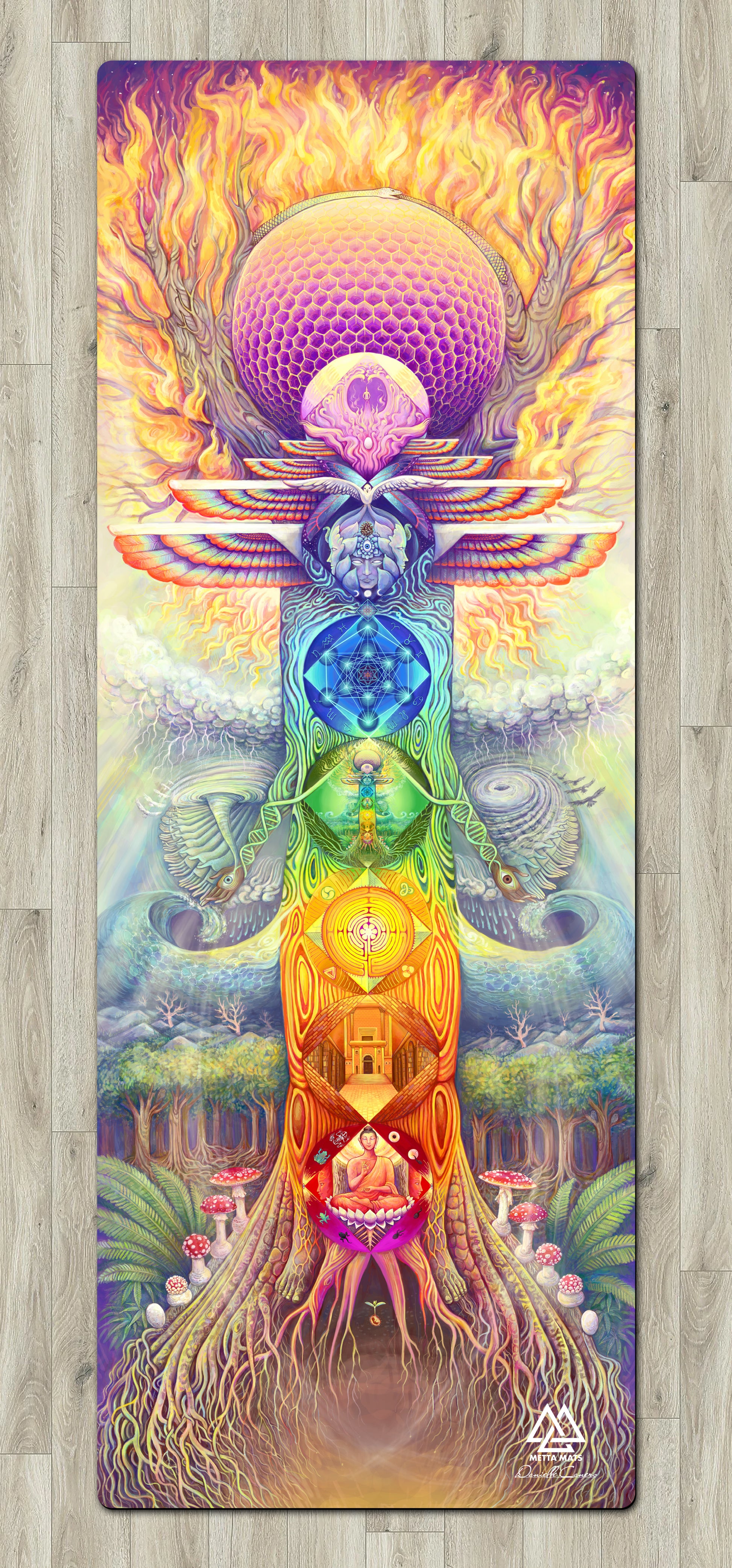This vibrant and intricate artwork depicts a fantastical tree that appears to belong to a magical realm. The tree, rich in detail and color, is set against a light brown platform that has a wood-like design. Starting from the bottom, the tree showcases a sprawling root system set against a tan background. Moving upward, the trunk is divided into various colorful segments, each representing different elements.

At the base, near the roots, the tree is tan with visible roots that seemingly delve underground. As the tree ascends, numerous fantastical scenes are engraved onto its trunk, each section colored distinctly. The lowest section near the base is red, showcasing images of buildings and possibly people. Above it, a yellow segment features a prominent large circle. Higher still, the tree trunk turns green, containing an image of a human figure with what appear to be arms protruding from it. This is followed by a blue section, adorned with some diamond shapes and sparks.

The topmost part of the tree opens into a large purple-colored globe, adorned with hexagonal patterns in purple, orange, and yellow. Flames of purple, orange, and yellow seem to erupt from this globe, culminating the tree’s vibrant display.

Surrounding this artwork is a frame that looks like lighter brown wood, almost gray in appearance, adding to its abstract yet organized design. Throughout the piece, there are splashes of numerous colors including purple, yellow, pink, blue, green, white, orange, red, and brown, creating a mesmerizing visual experience. The bottom right corner of the platform features a logo of three connected white triangles and some cursive text, adding a hint of mystery to this enchanting scene.